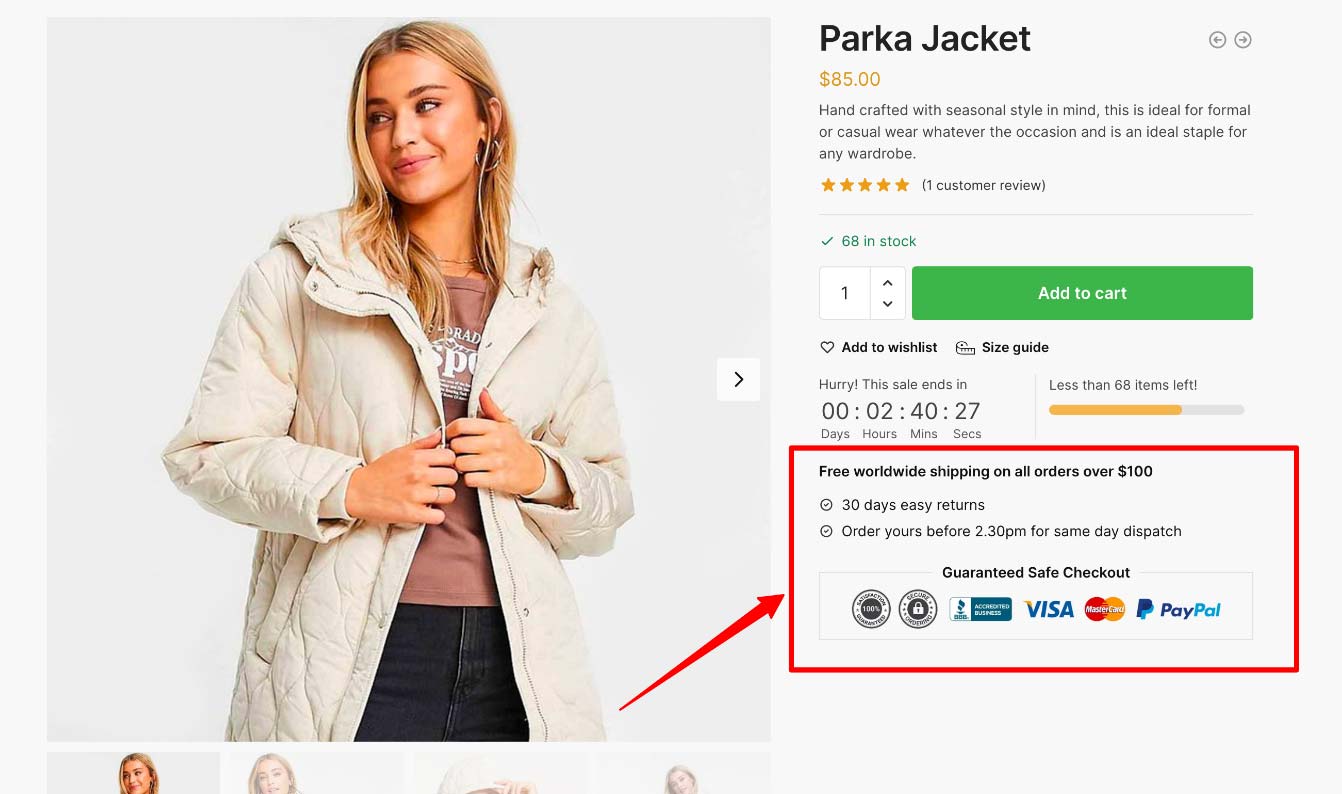This website advertisement features a captivating promotion for a stylish pinkish light parka jacket available for $85. On the left side of the ad, a woman models the long, quilted parka, looking slightly to the left with a subtle smile on her face. Her outfit pairs the jacket with a casual t-shirt and either blue jeans or a denim skirt, complementing her long hair.

On the right side of the advertisement, the headline prominently reads "Parka Jacket." Below this, the price is clearly stated as $85. The description highlights the jacket's handcrafted design, emphasizing its versatility for both formal and casual occasions, making it a must-have addition to any wardrobe. 

One glowing customer review, rated at five stars, is mentioned, along with the current stock count of 68 jackets. Potential buyers are prompted to select their desired quantity using the selection box, with an “Add to Cart” button conveniently placed to the right. 

A sense of urgency is created by a countdown timer indicating that the sale ends in two hours, 40 minutes, and 27 seconds, accompanied by a stock meter showing the rapidly decreasing availability. 

At the bottom, a rectangular box with a red outline offers additional incentives: "Free Worldwide Shipping on All Orders Over $100" and "30-Day Easy Returns." Customers are also encouraged to place their orders before 2:30 p.m. to ensure same-day dispatch.

Overall, the ad is designed to entice shoppers with limited-time offers and detailed product information, urging a quick purchase decision.